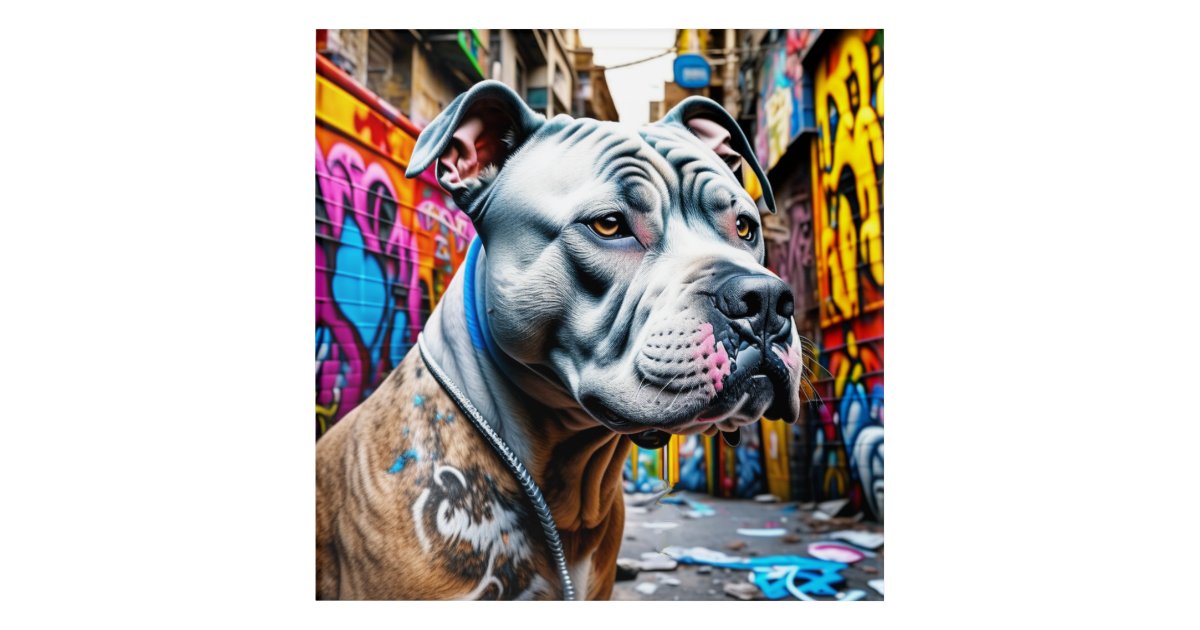The image is an AI-generated illustration of a pit bull with both a gray head and brown coat, accented with some blue speckles. The dog's forehead and cheeks are notably wrinkled, and it has distinctive pink and black splotches around its nose and mouth. An unusual detail is a silver cable or collar that appears to be embedded in or loosely hanging around its neck. The dog, which also has alert yet slightly flopped ears, is depicted sitting in a graffiti-covered alleyway. The walls on either side are adorned with vibrant pink and yellow graffiti, while the grayish ground is littered with debris. The alley appears narrow and enclosed by tall buildings.